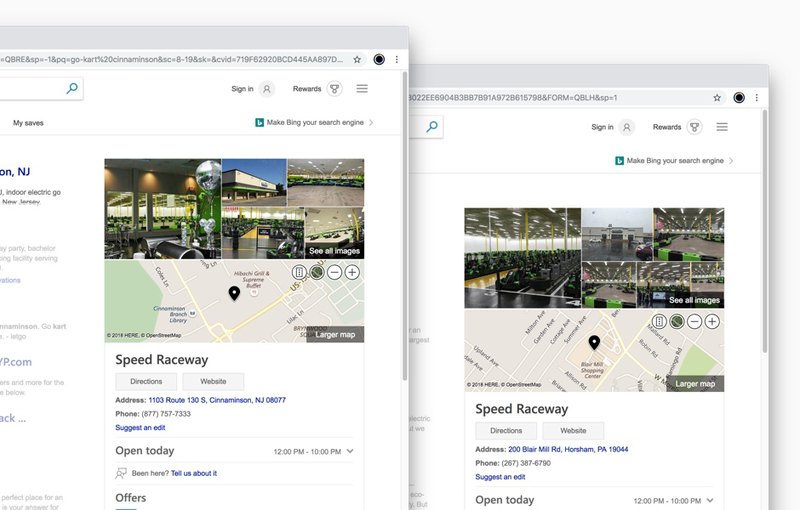Two overlapping screenshots depict a webpage header and search results for what appears to be a speedway or racing venue. The header includes a grey top bar featuring a web address bar with a grey star icon, a black circle icon, and three dots on the right side. Below this, part of a search bar with a grey magnifying glass is visible, followed by a white section. On the far right of the header, there are links labeled 'Sign up' and 'Rewards,' indicating a Microsoft Rewards page.

The left screenshot reveals partial search results for a location in New Jersey, including a speedway with various images: two outdoor scenes and three indoor ones. A map indicating the venue's location is shown, with the text "Speedway Race" or "Speed Raceway" along with clickable directions, a blue-hued address (which isn’t clearly readable), and a grey phone number. It also details operational hours, stating the venue is open today from 12 PM to 10 PM. Below this information, there's an option to suggest an edit, written in blue.

The right screenshot, although featuring nearly identical information, shows different images and a different phone number, revealing that there are two locations - one in New Jersey and the other in Pennsylvania. The variations in phone numbers and images suggest updates or differences between the two venues.